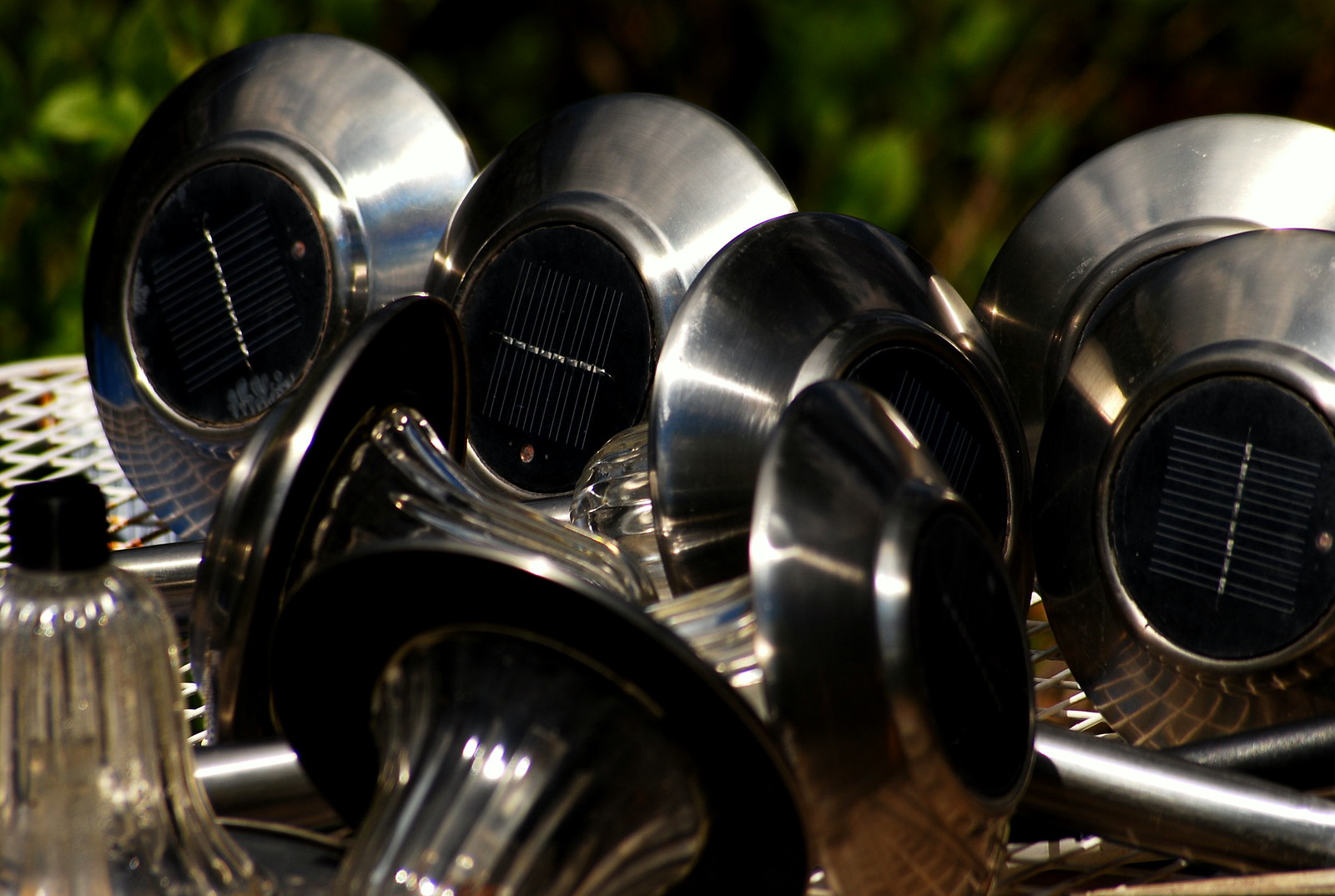The image captures a detailed close-up of a stack of approximately ten solar-powered landscape lights arranged haphazardly on a white metal wicker table, possibly made of painted wrought iron. These garden lights, clean and well-maintained albeit not new, feature silver rods designed to stick into the ground and semi-clear, ridged glass tops housing the light bulbs. Each top is capped with a black voltaic cell characterized by a silver line down the middle and wires crisscrossing in a circle. The background is slightly blurred, with hints of what might be trees and part of a mesh chair, enhancing the focus on the shining, bright stainless steel landscape lights ready for installation.